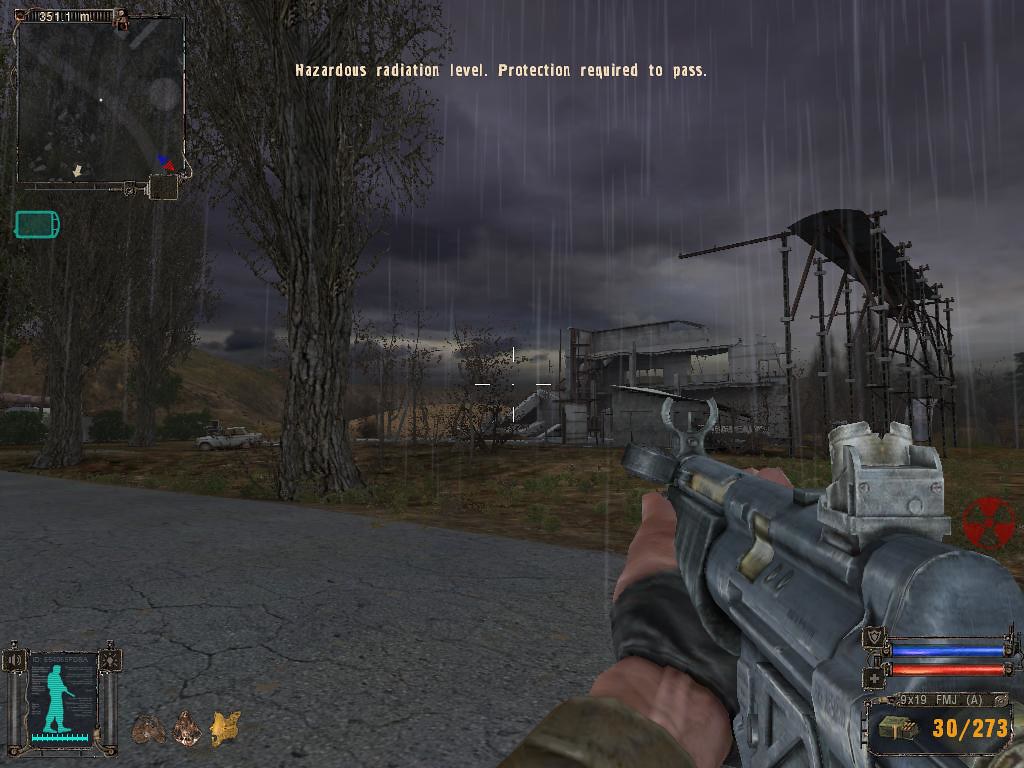This square-shaped image captures a moment from a gameplay scene. In the top-left corner, there is an in-game map, also square, featuring red and blue directional arrows at the bottom right. The map displays coordinates reading "351.1" at the top, while a message to the right states "Hazardous radiation level: Protection required to pass" in white text. At the bottom right of the image, a character's hand grips a gray rifle. The background reveals a dark gray and white sky, adding to the ominous atmosphere of the scene.